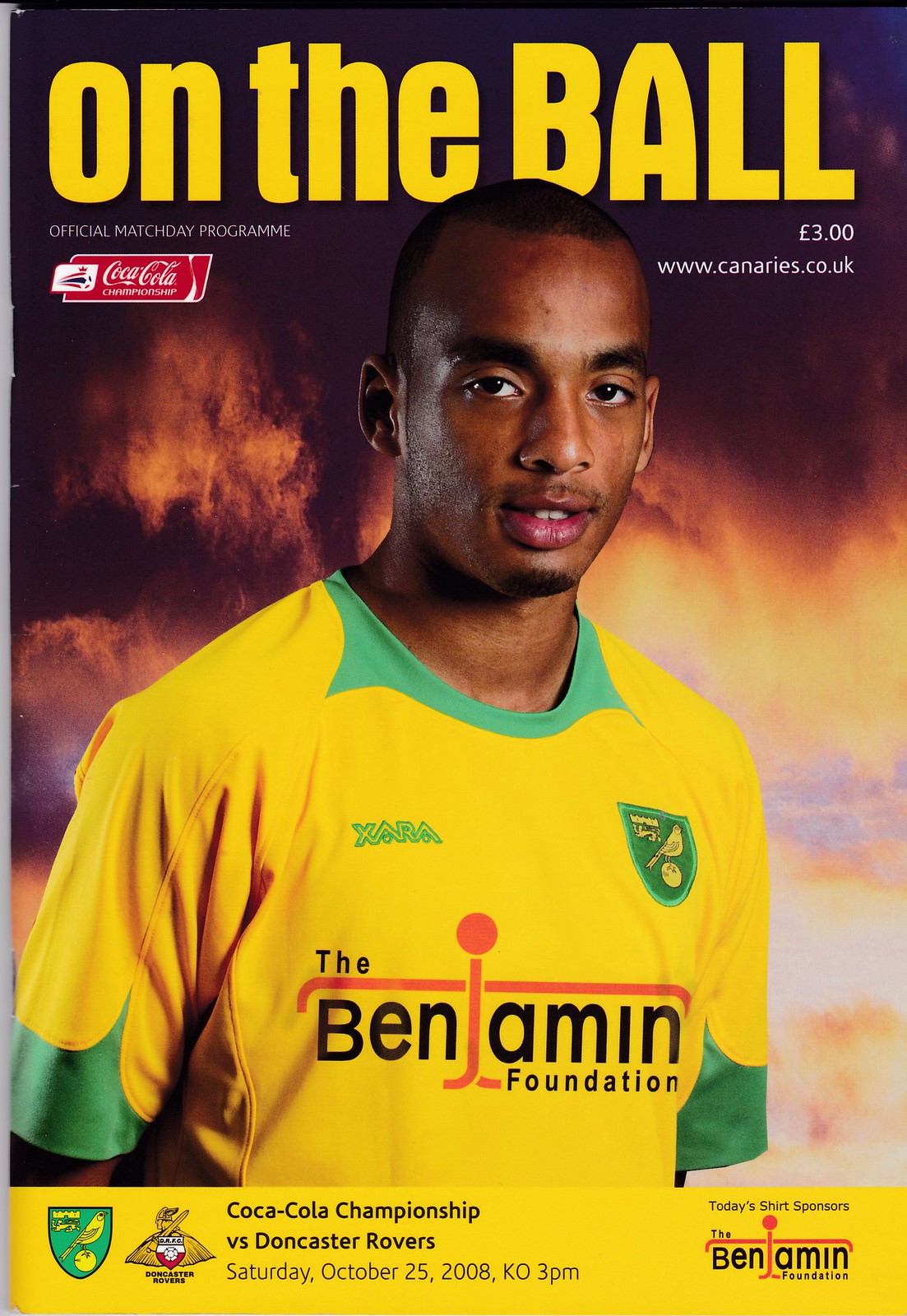The image depicts the front cover of an official match day program for a football game between the Canaries and Doncaster Rovers, dated Saturday, October 25, 2008, with a kickoff time of 3 PM. The background features a gradient from black at the top to fiery orangey-red hues. At the top, "On the Ball" is prominently displayed in bright yellow text. Below this, to the left, it states "Official Match Day Program" and features the Coca-Cola logo, while to the right, it shows the price as £3 and the website www.canaries.co.uk. The central image is of a young African American male with a shortly shaved head and a small beard, wearing a bright yellow sports jersey with green trim around the collar and sleeves. The jersey displays "The Benjamin Foundation." At the bottom of the cover, a yellow banner includes the text "Coca-Cola Championship versus Doncaster Rovers," alongside two logos. Additionally, the banner notes the match date and time. The bottom right corner mentions that today's shirt sponsors are The Benjamin Foundation.